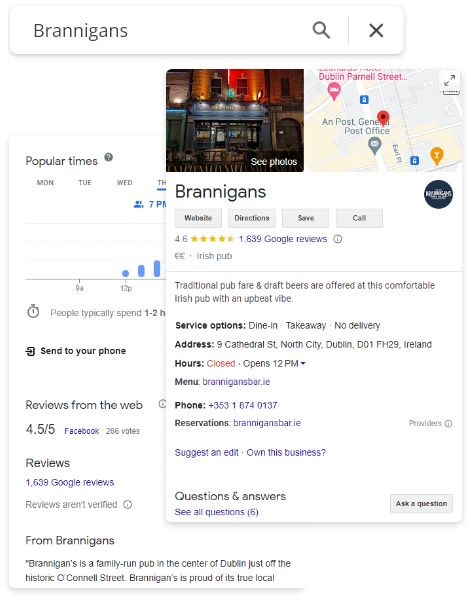The image displays a Google search results page for "Branigan's," a family-run Irish pub located at 9 Cathedral Street, North City, Dublin, Ireland. The search input clearly indicates "Branigan's." The page highlights that Branigan's offers traditional pub fare and draft beers in a comfortable setting with an upbeat vibe. Key service options include dine-in and take-away, but no delivery is available. The establishment's hours show that it is currently closed and will open at 12 PM. Further information includes the pub's menu available at branigansbar.ie and their contact phone number, +353 1 870 137. The description underscores Branigan's dedication to being a true local gem, situated just off the historic O'Connell Street in the heart of Dublin.